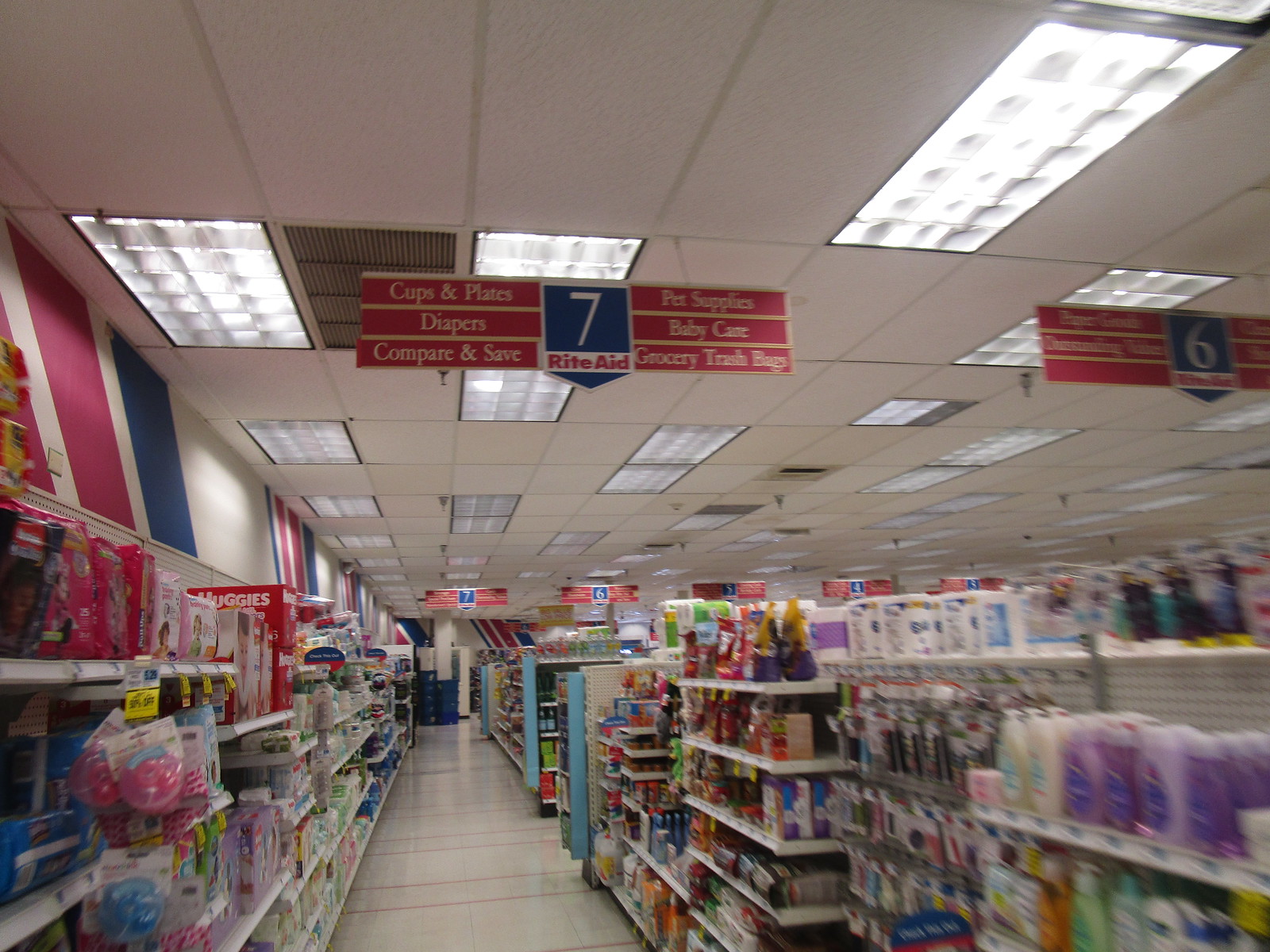The image captures the interior of a well-lit Rite Aid store. Prominently displayed is a red, rectangular sign indicating aisle number seven, where various items such as cups and plates, diapers, computers, compare and save deals, pet supplies, baby care products, and grocery trash bags are available. The store's ceiling is equipped with numerous elongated light fixtures that provide excellent illumination. In addition to aisle seven, a sign for aisle six can also be seen hanging from the ceiling. The shelves are stocked with a variety of products, and the white floor enhances the store's bright and clean appearance. The right-hand side of the image is slightly blurred, adding a dynamic element to the scene.